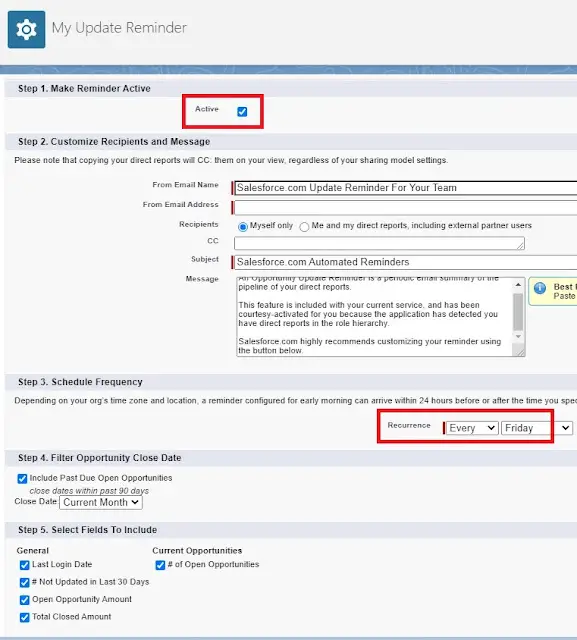This screenshot captures a detailed view of the configuration screen for an update reminder within a Work in Progress (WIP) system. The image focuses on the left side, revealing a step-by-step setup process. 

At the top, there's a settings icon, followed by the instruction title, "My Update Reminder." The first step is to activate the reminder, indicated by a red rectangle showing the activated box now turned blue from a click.

Step two covers customizing recipients and the message. The note specifies that copying direct reports will send them the same reminder regardless of sharing settings. The 'From' email address is pre-filled as "Salesforce.com Update Reminder for Your Team," with no secondary email address provided. The recipient field shows the user's cell phone, indicating that they want these reminders solely for themselves.

A "Copy and Close" option is visible, including a subject line reading, "Salesforce.com Automated Reminders." The message section suggests that several versions of the message have been typed and recommends pasting content to avoid errors.

Schedule frequency is set to every Friday, ensuring regular updates. Step four involves filtering opportunities based on their close date for the current month, and the user has chosen to include every field in the updates.

This setup reflects thorough preparation for receiving automated updates, ensuring timeliness and comprehensiveness in the provided information.